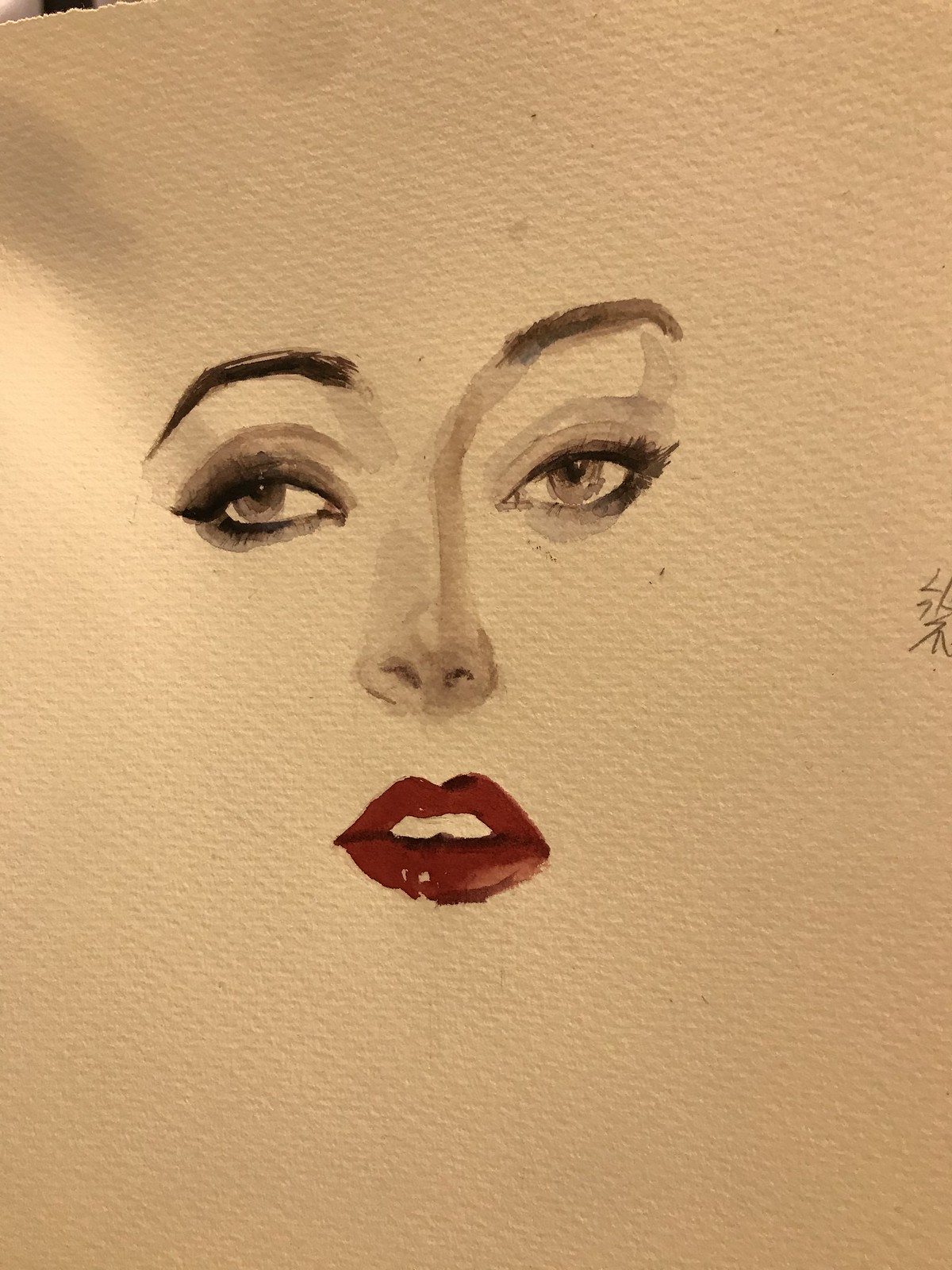A detailed painting on canvas features a woman's face without a defined outline, but with distinct facial features. The focus is on her eyes, nose, and mouth, with her lips painted a striking red. Her two prominent upper front teeth are visible, contributing to a detailed expression. Her nose and finely shaped eyebrows are clearly depicted. The woman appears to be wearing gray eye shadow, complemented by eyeliner and mascara on both the upper and lower lashes, enhancing the beauty of her light brown eyes. The eyeballs and pupils are meticulously painted, giving her a realistic gaze that is almost directed straight ahead, but slightly oriented towards the viewer's left.